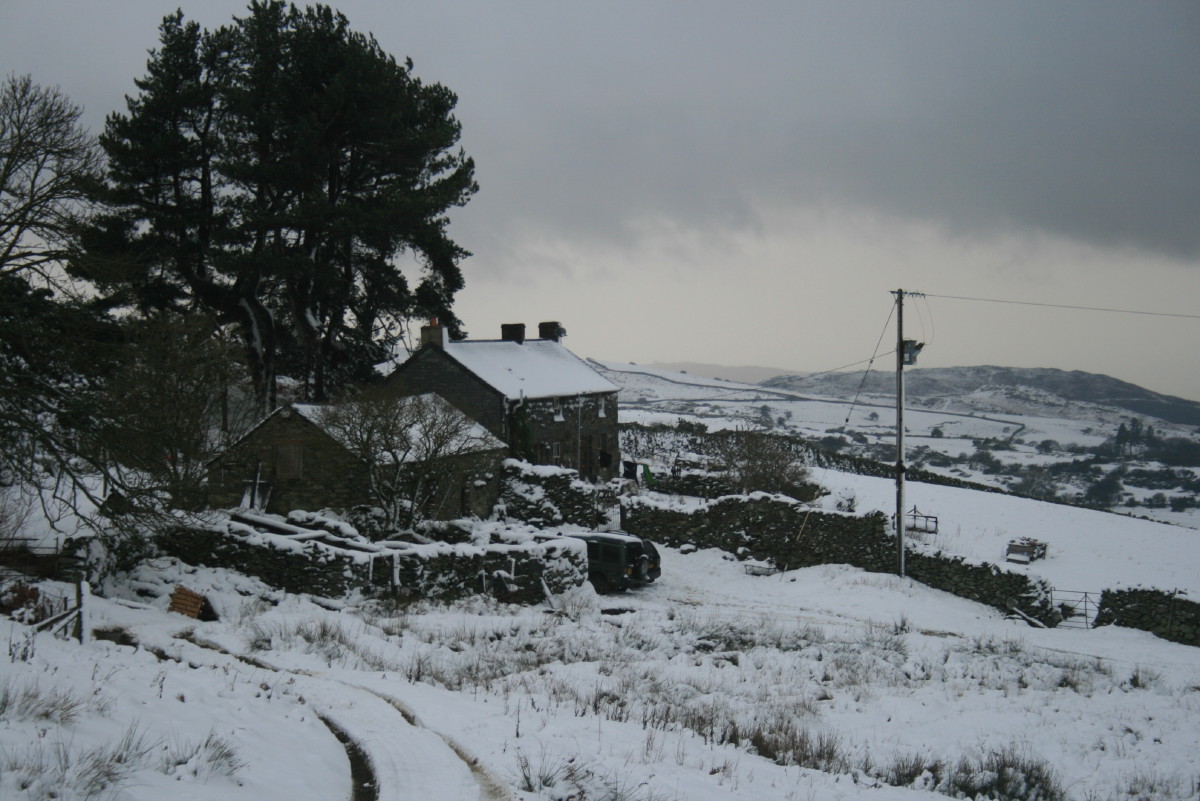A desolate, snow-covered homestead is depicted in this photograph, emanating a gloomy and timeless atmosphere. The overcast winter sky, dominated by thick gray clouds, casts a somber tone over the scene. The main structure, an older house likely built from stone or brick, prominently features three chimneys, suggestive of its historical roots. Attached to the house is a smaller substructure, perhaps a shed or garage, equally cloaked in snow. The entire property is encircled by a low stone wall, adding to its rustic charm.

In the front yard, an electrical pole stands as a solitary testament to modernity, with a power line extending towards the house. The ground is blanketed in fresh snow, betraying recent snowfall, and tire tracks carve through the icy terrain, leading to the back of a parked SUV. Surrounding the homestead, a serene landscape unfolds; tall pine trees loom behind the buildings, while to the right, tire tracks snake their way through the snow. Distant hills and an expansive open field stretch out towards the horizon, adding depth and a faint whisper of isolation to the scene.